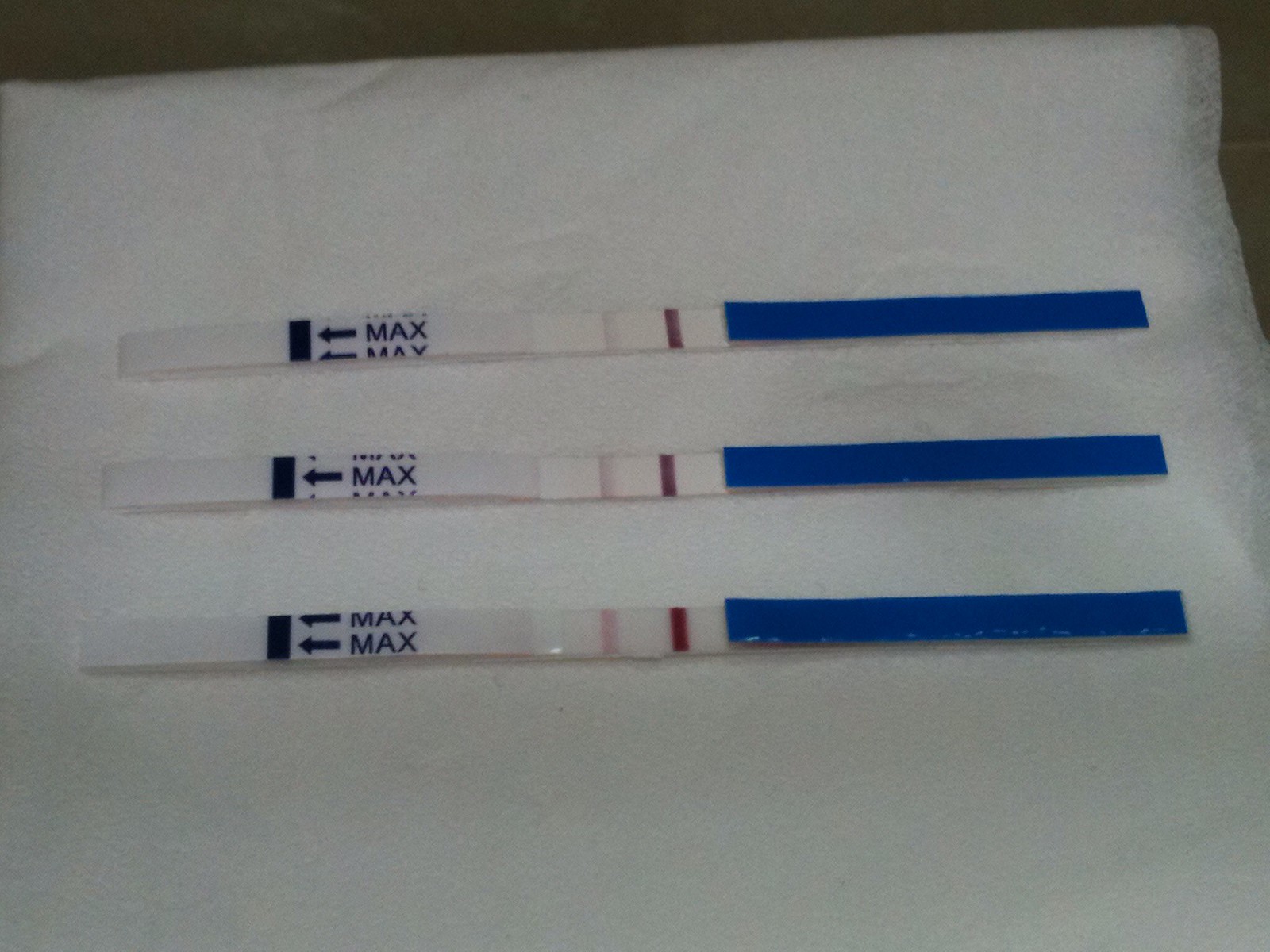The image features a background that resembles a white paper towel, napkin, or medical paper, with approximately an inch of black bordering along the top and slightly into the right corner. The focal point of the image consists of three similar long rectangular sections, each measuring about half an inch in height and about seven inches in length.

In the first rectangle, a vertical black line is positioned beside a blue arrow pointing left, accompanied by the text "M-A-X" in blue letters. Moving roughly four to five inches to the right, there is a series of vertical lines: one faintly pink, followed by a burgundy line, and then a small white square. The remaining portion of this rectangle is filled in blue.

The second rectangle directly below mirrors the first exactly.

The third rectangle at the bottom is nearly identical, but with two blue arrows pointing left and the full "M-A-X" text appearing twice. Unlike the first two rectangles, which only show the tips of the "M-A-X" text, this one displays the entire word clearly.